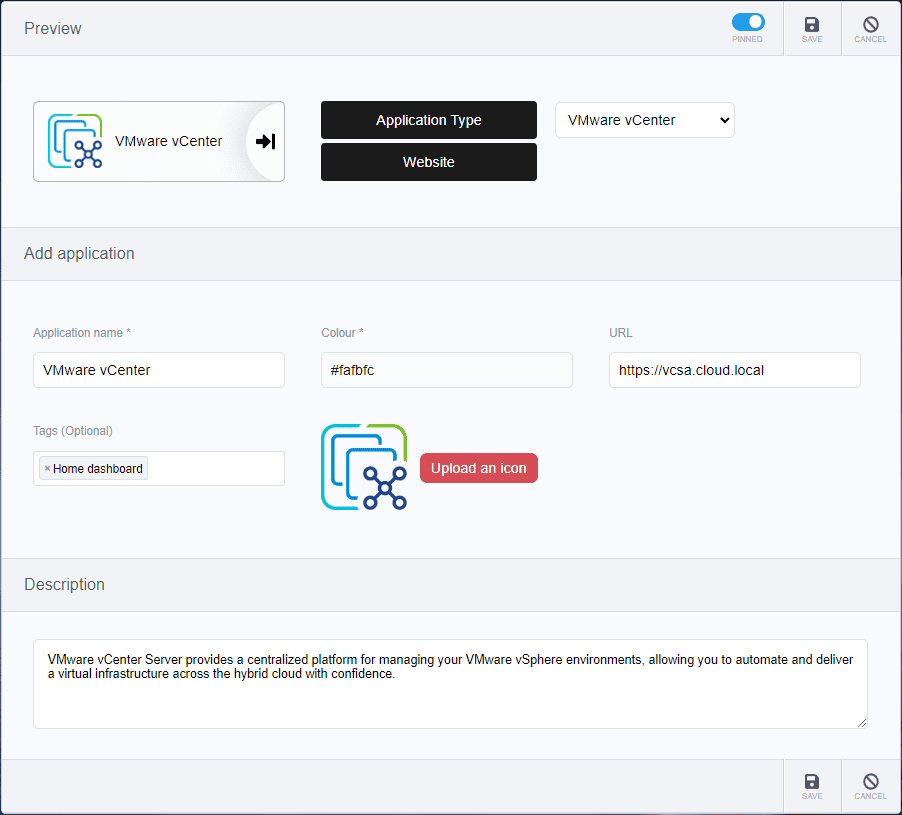This is an image of what appears to be the VMWare vCenter application interface. The top of the window is not visible, leading to some uncertainty about the exact application. In the top left corner, there is a "Preview" label accompanied by a sliding switch button labeled "Pinned," resembling the switch buttons commonly found on mobile devices. This switch has a circular toggle within a rounded rectangle.

Below the "Pinned" switch, there are "Save" and "Cancel" buttons, represented by a floppy disk icon and a circle with a strikethrough, respectively. A prominent button labeled "VMWare vCenter," with a logo next to it, is also present. The logo consists of three rectangles and a cross made out of circles, with the largest rectangle being blue and green and the others blue.

Further down, there are options for "Application Type" and "Website," both in black text. Other details include a dropdown menu labeled "VMWare vCenter," an "Add Application" button, and fields for "Application Name" (VMWare vCenter), "Color" (#FAFBFC), and "URL" (https://vCSA.cloud.local). Additionally, there are optional tags listed as "Home" and "Dashboard," along with a larger version of the VMWare vCenter icon seen earlier.

The next section features an "Upload an Icon" button. At the bottom, there is a description stating, "VMWare vCenter Server provides a centralized platform for managing your VMWare vSphere environments, allowing you to automate and deliver a virtual infrastructure across the hybrid cloud with confidence." The bottom right corner of the interface also contains the same "Save" and "Cancel" buttons as seen in the upper right.